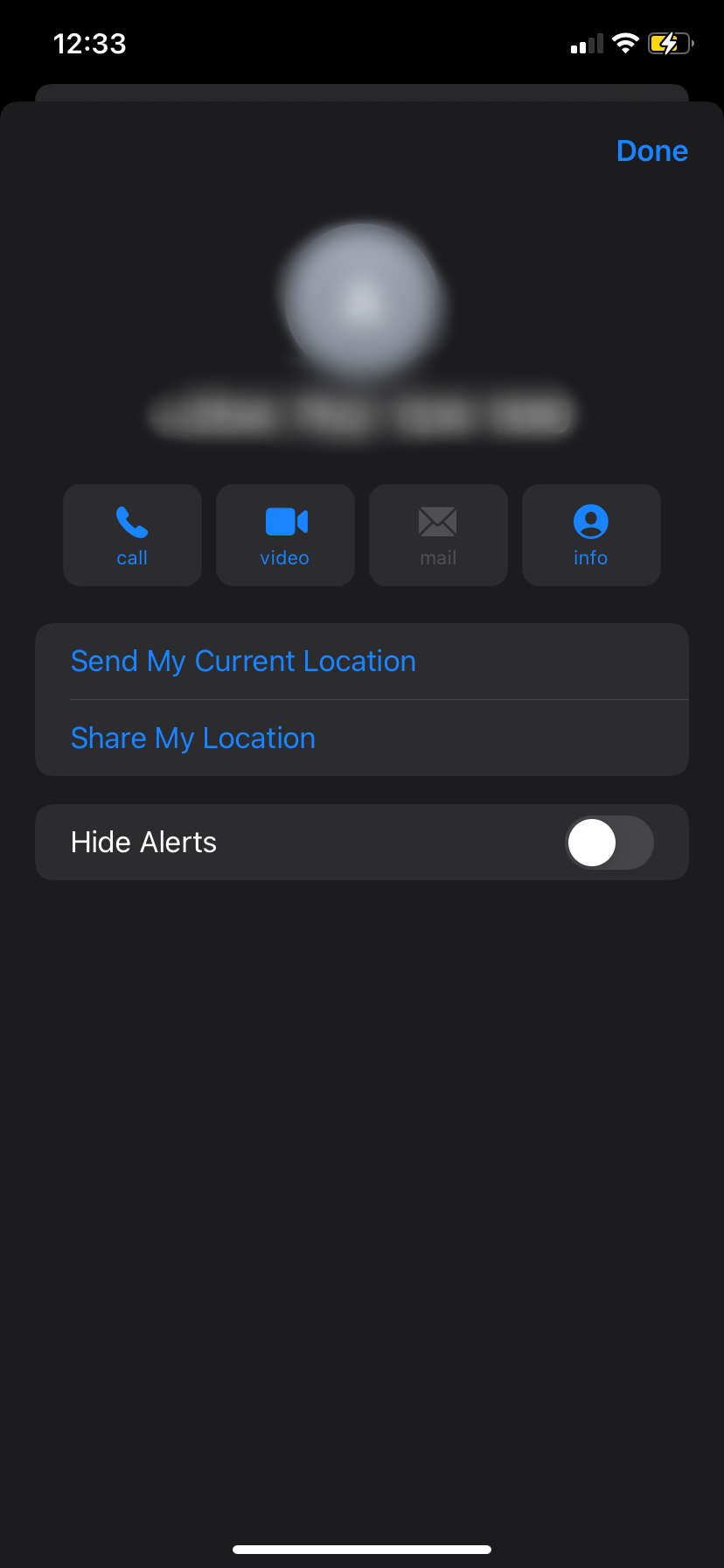The image is a screen capture from a cell phone displaying a contact in the phone's contact list. The status bar at the top of the screen shows a charging battery with approximately 50% life, a Wi-Fi connection, and two bars of cellular service. The time displayed on the phone is 12:33. 

The background of the screen is black. In the upper right corner of the screen, there is a blue "Done" button. The central part of the screen, where the contact's profile picture and information would normally be visible, is completely blurred out, obscuring the identity of the contact. 

Below the blurred section, there are four buttons arranged horizontally: a blue "Call" button, a blue "Video" button, a grayed-out "Mail" button, and a blue "Info" button. Directly below these buttons, in blue text, is an option that reads "Send My Current Location." 

A thin gray line separates this option from another blue-text option below it, labeled "Share My Location." Further down, there is a section titled "Hide Alerts" with a toggle button that is currently unchecked. 

At the very bottom of the screen, a wide, horizontal white bar extends from the center towards the edge, likely representing the home button or navigation bar commonly found in modern smartphones.